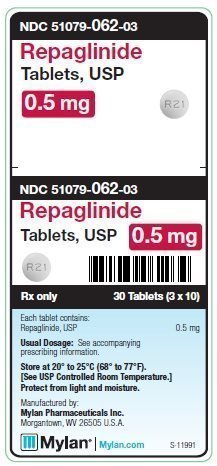A detailed caption for the described image:

“The image displays the user interface of a phone showcasing detailed labeling information for a pharmaceutical product. The outer border of the UI is a greenish-gray color, enclosing all elements within. Inside this border, there is a dark black box. At the top of this black box, a black bar prominently displays the text 'NDC 51079-062' in large lettering, accompanied by '0.003'. Beneath this, 'REPAGLINIDE' is written in red, with additional labeling indicating 'tablets USP' and dosage '0.5 Milligrams' in smaller text. There is also an illustration of a tablet labeled 'R21' (not 'RZ1' as initially mentioned), set against a white background. The '0.5 milligrams' text is enclosed within a red box, and the red 'REPAGLINIDE' text is reiterated. 

Below this section, two small horizontal lines extend from the left and right sides of the black box. Moving further down, another black border features the text 'NDC 51079-062-03', with '062' notably larger. Again, 'REPAGLINIDE' is written in red, followed by 'tablets USP' and '0.5 milligrams' in a red box. The depiction of the tablet labeled 'R21' appears once more, accompanied by a barcode.

Further details include 'Rx only for prescription on prescription only,' specifying '30 tablets 3 times 10.' Additional instructions detail each tablet containing 'Repaglinide USP 0.5 milligrams,' usual dosage guidelines, storage conditions of '20 to 25 degrees Celsius (68 to 77 degrees Fahrenheit),' and advisories to protect from light and moisture. Manufacturer information is provided: 'Mylan Pharmaceuticals Inc., Morgantown, West Virginia, 26505 USA.'

At the bottom left of the screen is the Mylan icon, characterized by an aqua blue color and enclosed within a black box, followed by a horizontal line and the URL 'Mylan.com' in aqua blue text. Finally, the bottom right of the screen displays 'S-11991.'"